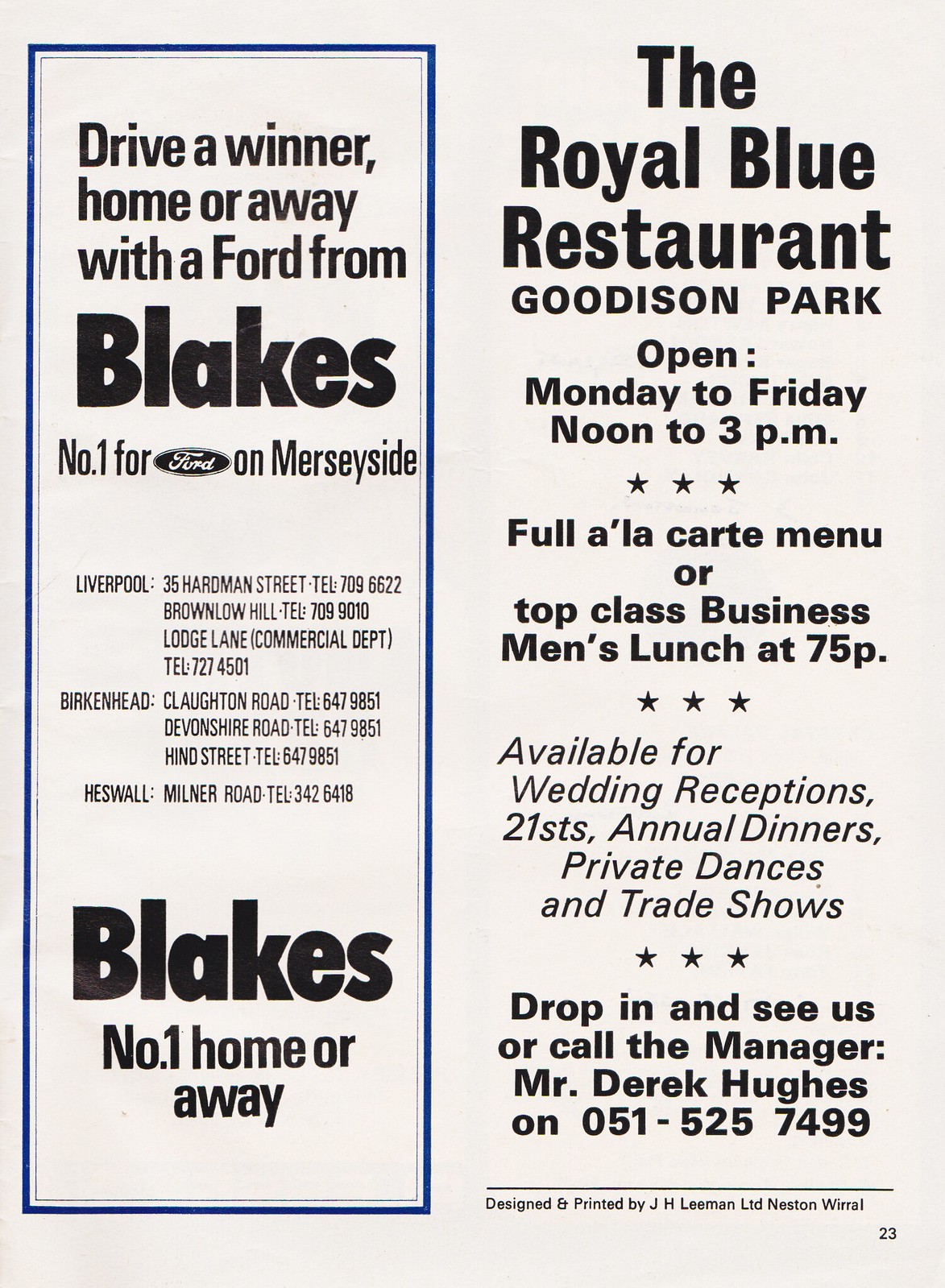This image is a scan of a page from a magazine or program booklet, indicating it's part of a larger publication, as evidenced by the page number "23" in the lower right corner. The page features two advertisements juxtaposed against a white background, with all text in black.

On the left side of the page is a vertically aligned ad for Blake's Ford dealership, bordered by a thin blue line forming a rectangle. The ad prominently displays the slogan, "Drive a winner home or away with a Ford from Blake's," and highlights Blake's as the number one Ford dealer on Merseyside. The ad lists several dealership locations along with their contact numbers:
- Liverpool: 35 Hardman Street, TEL 709-6622; Brownlow Hill, TEL 709-9010; Lodge Lane, Commercial Department, TEL 727-4501
- Birkenhead: Claughton Road, TEL 647-9851; Devonshire Road, TEL 647-9851; Hines Street, TEL 647-9851
- Heswall: Milner Road, TEL 342-6418.

On the right side, there's an advertisement for the Royal Blue Restaurant at Goodison Park. This ad details the restaurant's operating hours and menu options: open Monday to Friday, noon to 3 p.m., offering a full à la carte menu or a top-class businessmen's lunch for 75p. It also mentions that the restaurant is available for wedding receptions, 21st birthday parties, annual dinners, private dances, and trade shows. The ad encourages readers to "drop in and see us" or contact the manager, Mr. Derek Hughes, at 051-525-7499.

The page closes with a note indicating that it was "designed and printed by J. H. Lehman, Limited, Neston, Wirral," marked by a separating black line.